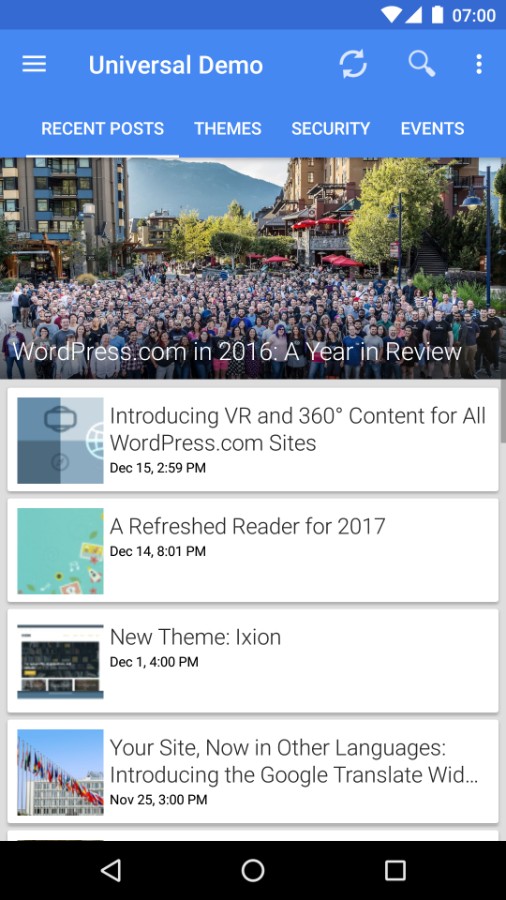This screenshot showcases an old iPhone capture of a section within the WordPress app. Dominating the top of the screen is a large blue header, prominently displaying "Universal Demo" on the top left in white text. Adjacent to this text, aligned to the right, are three icons: a refresh icon, a magnifying glass icon for search, and a vertical ellipsis icon indicating additional options.

At the lower part of the header, there are several navigation categories, all in capital letters and white font: "CATEGORIES," "RECENT POSTS," "THEMES," "SECURITY," and "EVENTS."

Beneath the header, a significant portion of the screen is occupied by a large company group photo. At the bottom left corner of this image, text reads "WordPress.com in 2016, a year in review."

The main content area below this image features a vertical list of horizontal stories or ads. Each entry comprises a thumbnail image on the far left, followed by the title of the story and the date posted in small black letters underneath the title. The topmost story is titled "Introducing VR in 360 Content for all WordPress.com sites."

Lastly, a scroll bar is visible on the far right side of the app screen, indicating that there is more content to explore further down.